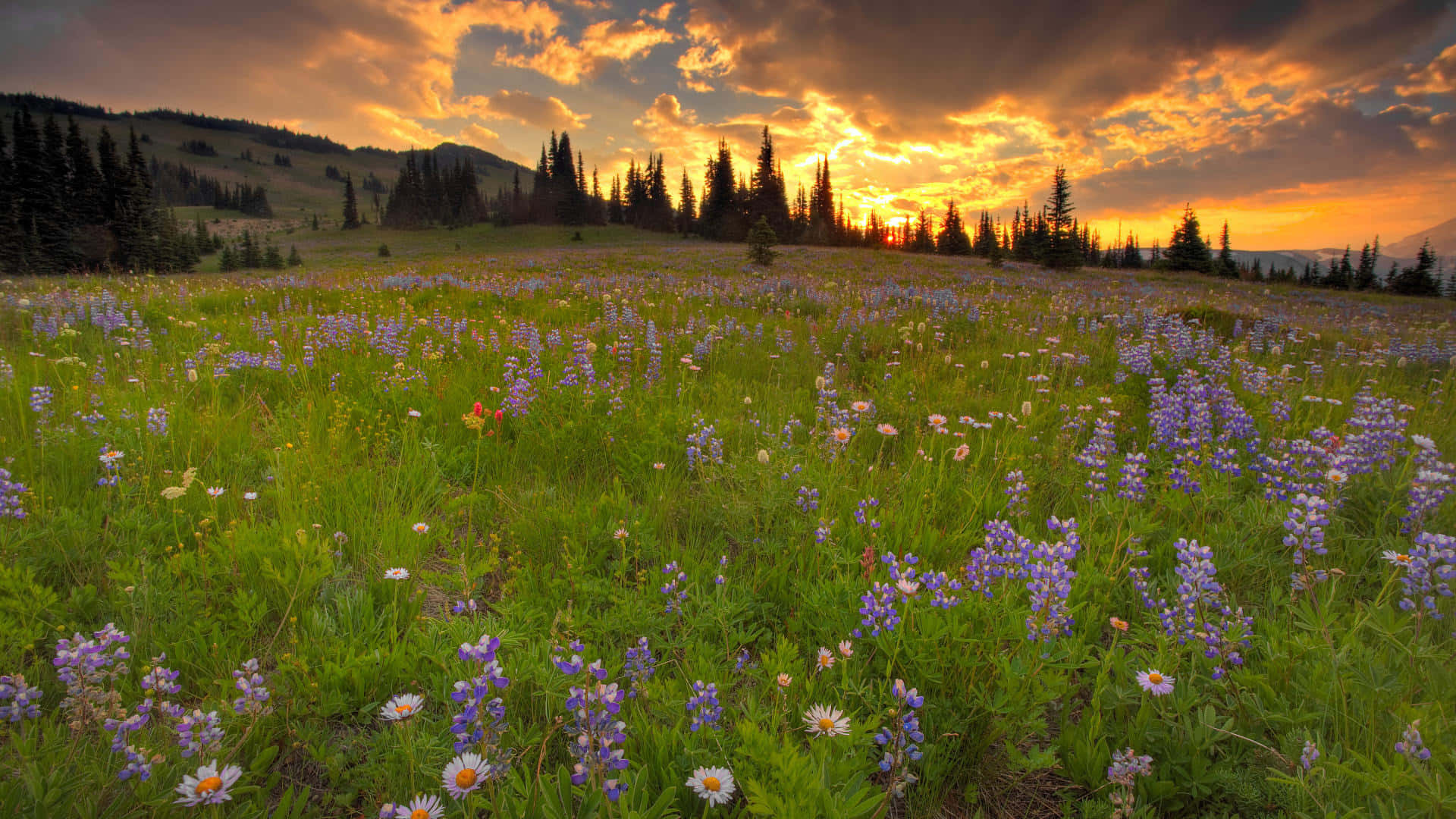The image captures a breathtaking meadow filled with a variety of vibrant flowers and lush green grasses. The field, blanketed predominantly by small purple flowers with white centers, is interspersed with white daisies featuring yellow centers and some long-stalked blue flowers. There are also occasional red flowers adding a splash of color amongst the greenery. The scene is bathed in the warm hues of a setting sun, which casts a golden-orange glow across the landscape. Thick, puffy clouds in shades of purple, pink, and blue dominate the predominantly blue sky, making for a dramatic backdrop. To the right-hand side, rows of tall, conical pine trees stretch towards the horizon, while on the left, a grassy hill dotted with sporadically placed trees ascends gently. The meadow extends up past the middle of the image, merging seamlessly with the picturesque sky, creating a harmonious blend of nature’s beauty.